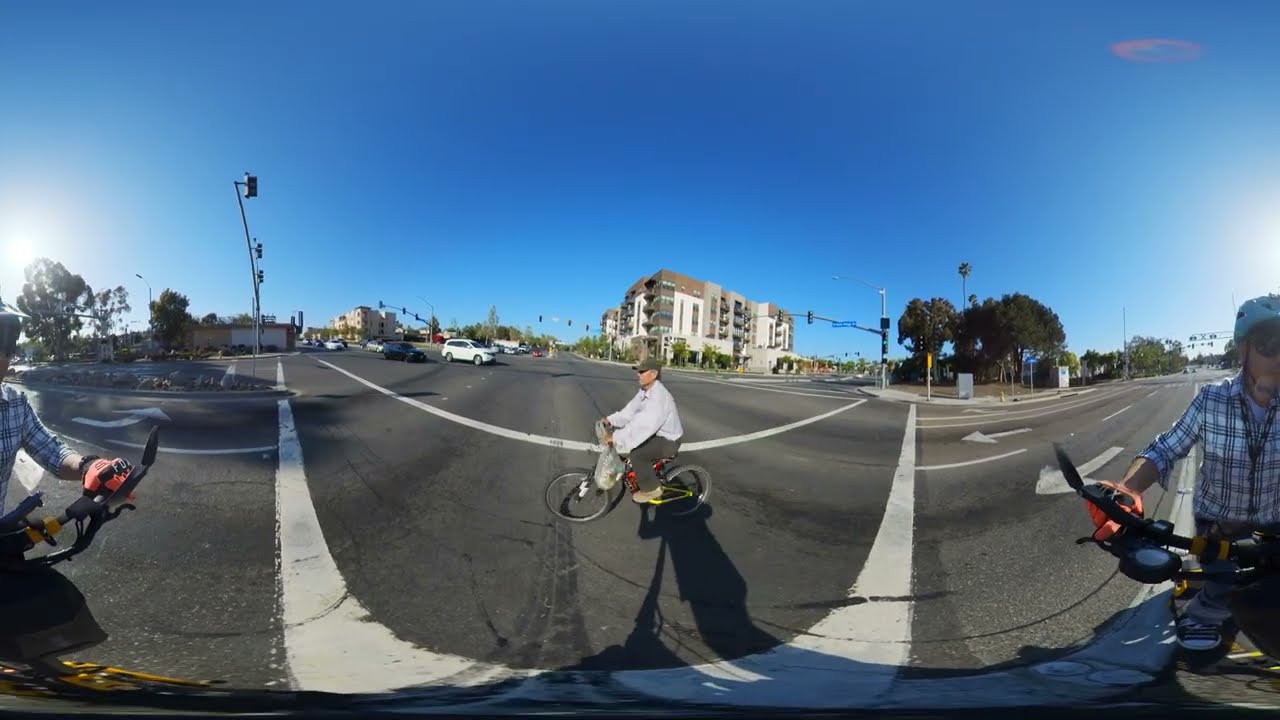This panoramic photograph, slightly warped due to its stitched composition, captures a bustling street intersection on a bright, cloudless day. At the center, a man in his 40s or 50s is riding a bicycle through a pedestrian crosswalk, heading towards the left. He is dressed in a white button-down shirt, gray khakis, and a gray ball cap, with a plastic bag hanging from his handlebars. Flanking the image's far left and right edges, the same man appears again, each time partially cut off due to the panoramic effect, this time wearing a gray and white plaid button-down shirt, a helmet, and sunglasses. He holds a red object, possibly a bike accessory. The background features a mix of high-rise condominium or office buildings, about four stories tall, and various cars, including a white and a blue vehicle, traversing the intersection. Street lights and a few median trees add to the urban setting. There is a noticeable white building, possibly an apartment complex, centrally situated in the background, and a prominent highway with marked lanes in the foreground. The entire scene is completed with a clear blue sky and the dynamic activity of the town intersection.